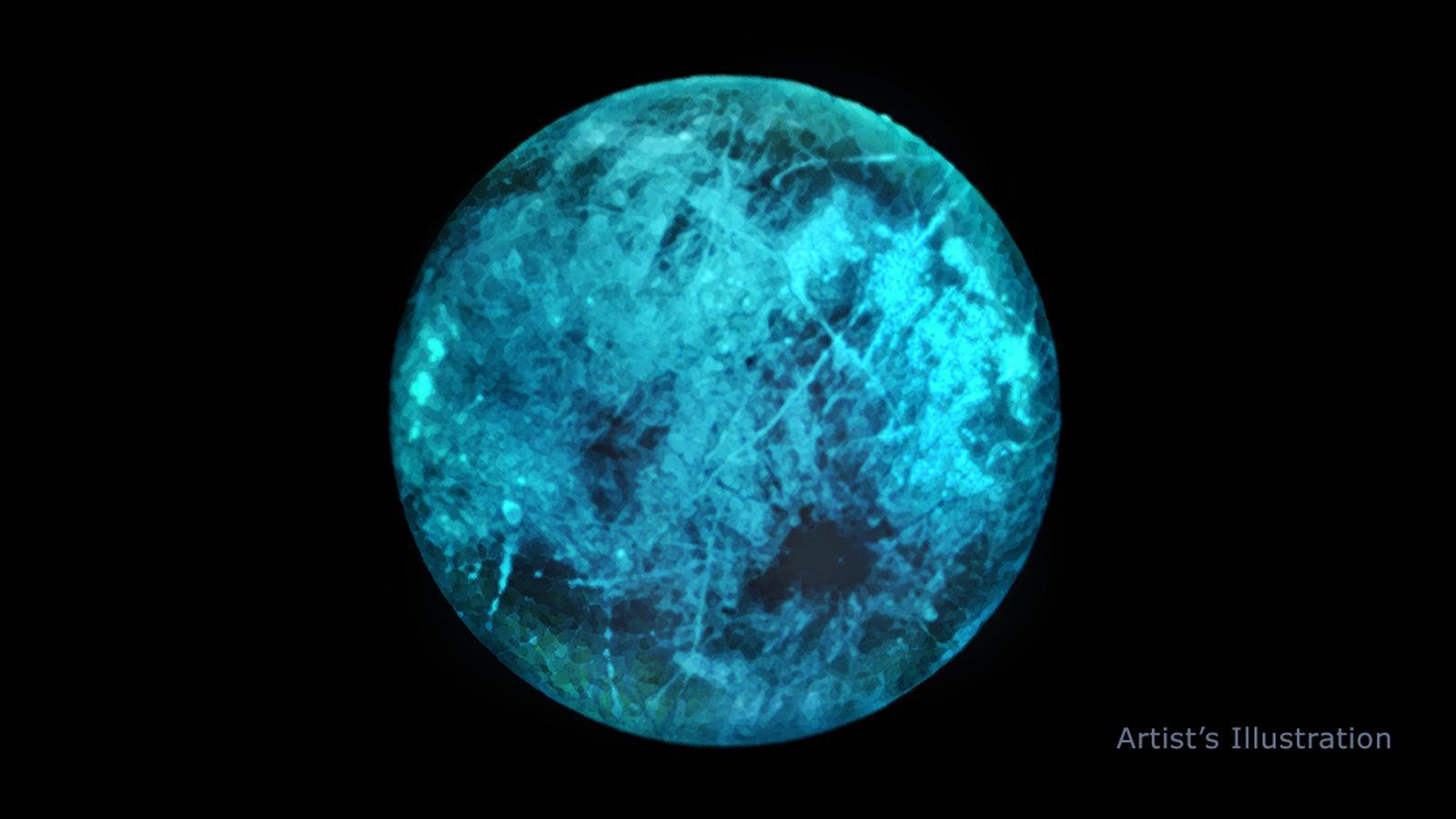This is a highly detailed artist's illustration set against a solid black background, depicting a close-up of a round celestial body, which could be interpreted as either Earth or the Moon. The planet is rendered in an array of blues, ranging from light to dark aqua shades, with no key provided to interpret these colors. The entire one side of the globe is shown, suggesting that the darker blue tones might represent oceans, while the lighter ones could signify land, although this is left ambiguous. The image is brightly lit, creating stark contrasts that emphasize its features, and takes up at least half of the rectangular frame. In the bottom right corner, there is a text that reads "artist's illustration," confirming the creative nature of the depiction.